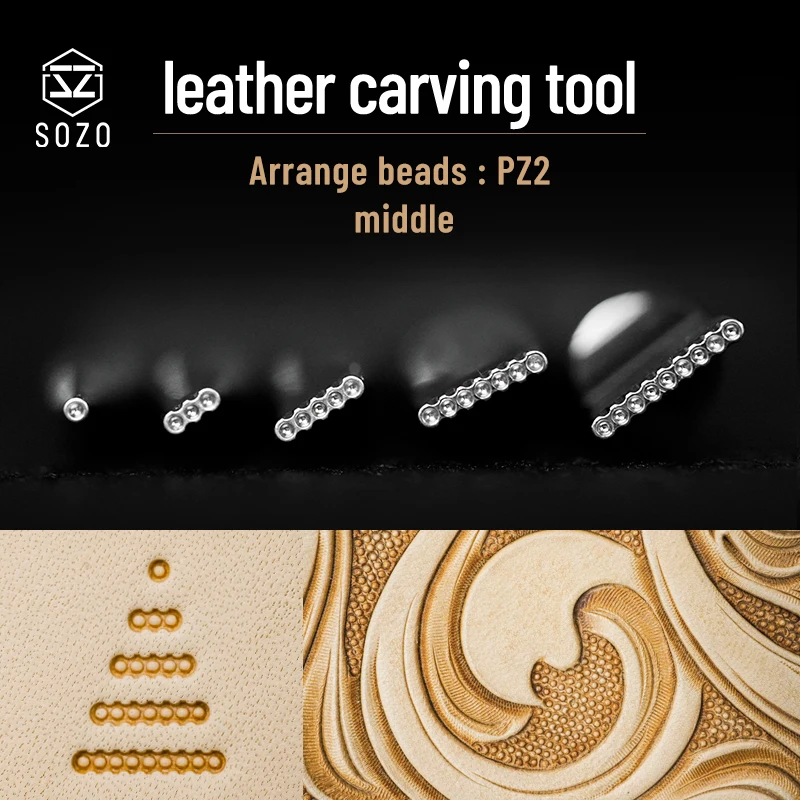The image is an advertisement for a leather carving tool by the company SOZO, featuring their unique logo with an 'S' and 'Z' facing each other. The top of the image has a black background with white text that reads "Leather Carving Tool," followed by an underline and the phrase "Arrange Beads: PZ to Middle." The top half showcases silver-tone tools, each designed to create specific bead patterns: one bead, three beads, five beads, seven beads, and nine beads, arranged in increasing order.

The bottom half of the image, which has a light tan and beige swirly background, illustrates the tool in action on a piece of very light-colored, almost ivory leather. On the left side of this section, the beads are arranged to form a pattern reminiscent of a Christmas tree, with one bead at the top, followed by lines of three, five, seven, and nine beads. The right side displays an artistic rendition of the swirly design, showing how these tools can be used for detailed and aesthetically pleasing leather carvings. The advertisement highlights both the precision and the artistic versatility of the SOZO leather carving tool set.